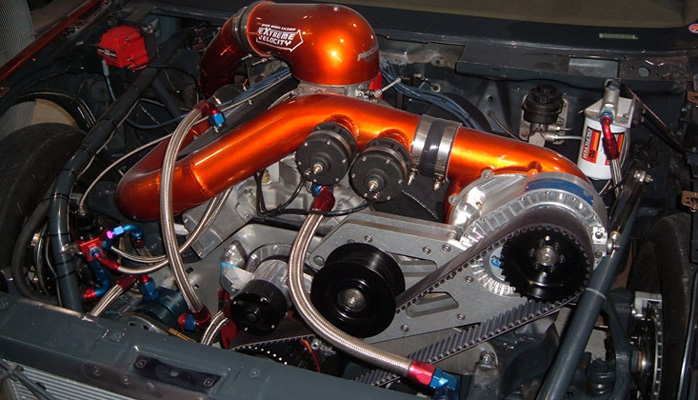This image showcases a close-up view of the engine bay of a high-performance vehicle, possibly a race car. The engine is prominently silver with a colorful assortment of components. The gray timing belt and black cylindrical pulleys are centrally featured, with braided aluminum hoses that have red and blue fittings. Bright orange aluminum exhaust pipes streak vibrantly across the top and towards the back, catching the eye. The engine bay also contains various black and silvery cables, a white oil filter on the upper right, and an oil dipstick. A small brake booster is visible, along with a hint of a roll cage surrounding the motor. The front grille is barely visible at the bottom edge of the frame. The hood is popped, revealing the gray exterior of the car and a faint glimpse of the beige dashboard and windshield at the top. Overall, the image highlights the intricate details and the colorful complexity of a high-performance engine.